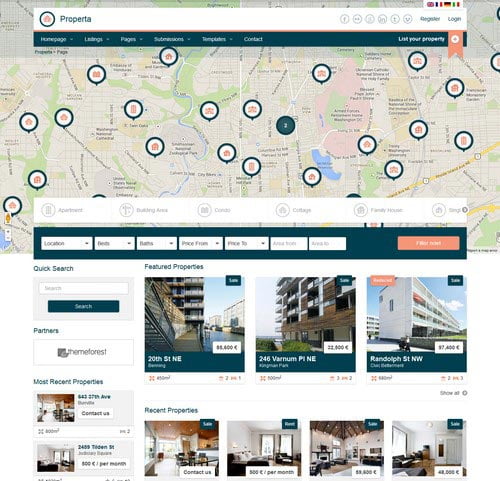This image showcases a detailed webpage from a property search website named Properta. Dominating the screen is a large, interactive map dotted with numerous circles, each representing a property listing. Most of these circles contain gold icons, with one standout dark green circle. The map also features white streets and a blue river flowing through the area.

Beneath the map, there's a section likely dedicated to hotel listings, including a location input field. Various drop-down menus are positioned nearby, allowing users to specify search criteria such as price. An orange box on the right side of the screen probably serves as a call-to-action button. Below this, the site displays actual photos of apartments or hotels along with recent property listings, providing a glimpse into different interior spaces.

On the left-hand side of the page, a "Quick Search" feature includes a search bar and a button to initiate the search. Additionally, the sidebar mentions partnerships and lists the two most recent property entries, ensuring users can quickly stay updated with the latest offerings.